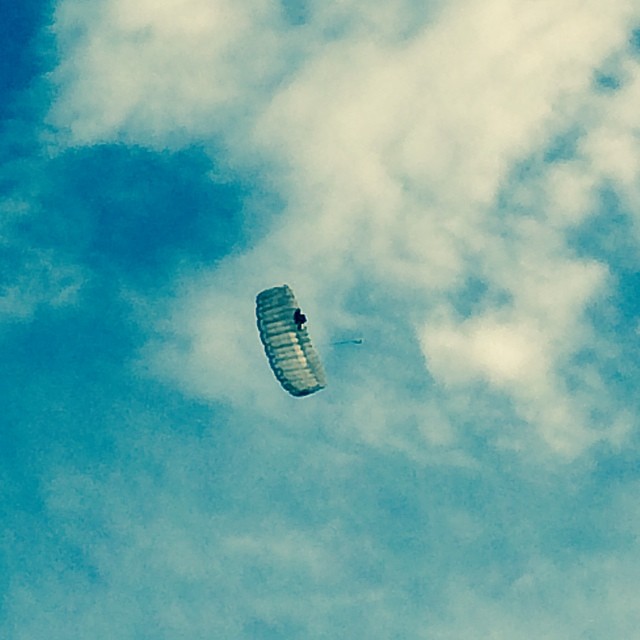In this captivating photo, the vast blue sky dominates the background, tinged with darker blues in the top left and dotted with white to gray clouds on the right. At the heart of the image, a paraglider, sporting a long rectangular parachute, elegantly unfurls against the serene expanse. The canopy, appearing slightly grayish with hints of green, catches the wind, revealing its underside to the viewer. Suspended beneath, a tiny black speck indicates the presence of a human, barely discernible at this distance. The scene is completed with faint strings trailing from the parachute, blending into the expansive horizon.